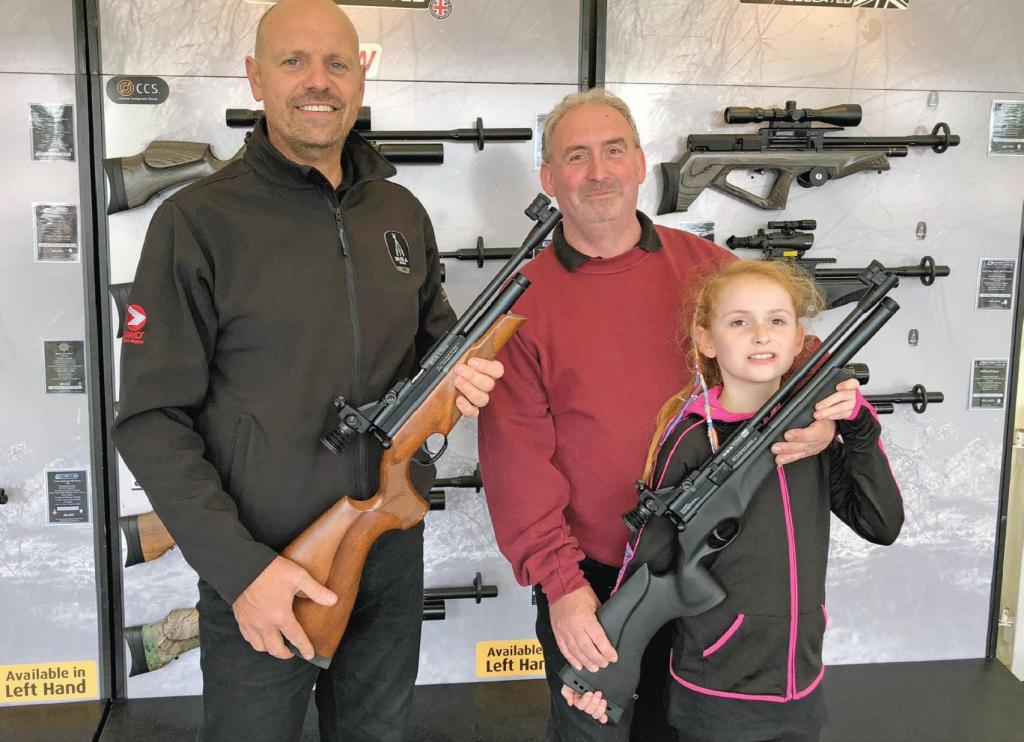The photograph captures a scene inside a gun store, where two middle-aged men and a young girl are posing in front of a display wall filled with various rifles. The man on the left is bald, dressed in a black zip-up jacket and black pants, and is smiling at the camera while holding a rifle that features a wooden stock and a black barrel. To the right, a man with gray hair and a slight five o'clock shadow is wearing a red sweatshirt over a black collared shirt. He stands behind a young girl with red braided hair, who is dressed in a black zip-up hoodie with pink trim. The girl, also focused on the camera, is holding a matte black rifle, with the man in the red sweatshirt assisting her grip. The background showcases an array of rifles on racks, adding to the gun store ambiance, though the exact details on the sign behind them remain obscured by their presence.